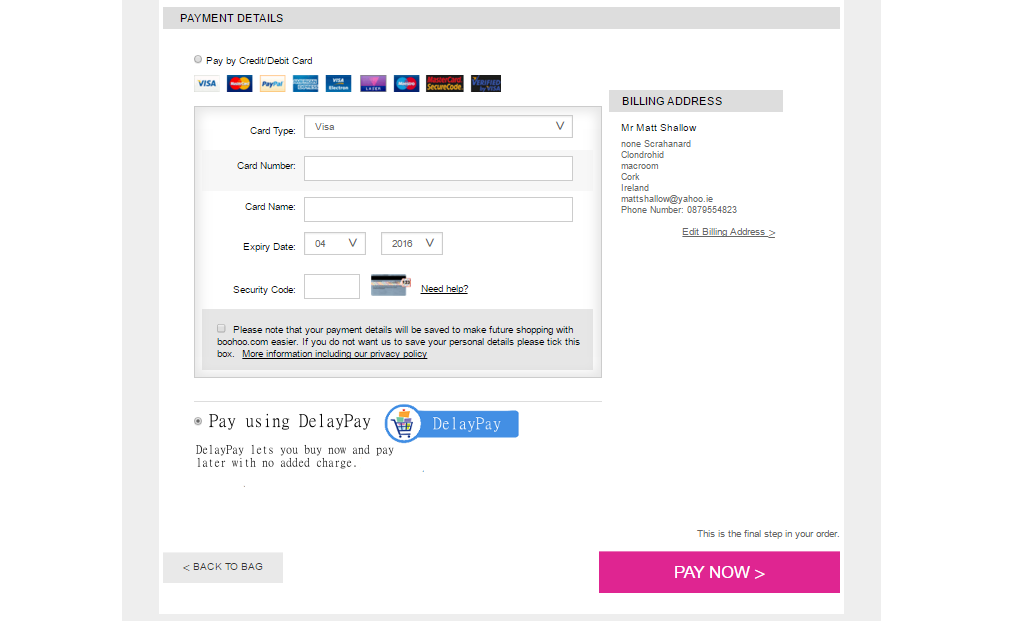The screenshot captures a payment page, characterized by a clean, organized structure surrounded by a gray border. At the top-left corner within this border, the text "Payment Details" is prominently displayed in black.

Central to the design, the white background hosts the primary interactive sections. A rectangular gray box is situated in the upper left corner of this white space, where it prompts users with the instruction "Pay by credit/debit card." Adjacent to this prompt is a horizontal array of logos representing various credit card companies, providing visual cues for acceptable payment methods.

Below this section is a form for entering payment information, offering fields for card type, card number, cardholder name, expiry date, and security code. At the bottom of this form, a cautionary note informs users that their payment details will be stored to streamline future transactions on boohoo.com. It also provides an option to opt out by checking a designated box, along with a reference to the company's privacy policy for more information.

To the right of the payment details box, the user’s billing address is displayed, indicating the details for Mr. Matt Shallow and Nunn Sarah Hannon. Although some lines are illegible, it specifies that the address is in Ireland and includes an unreadable email address and phone number.

At the bottom of the page, an alternative payment option, "Delay Pay," is described. This option allows users to buy now and pay later without additional charges.

The page concludes with a purple rectangular button in the lower right-hand corner, featuring the prominent call-to-action text "Pay Now" at its center.